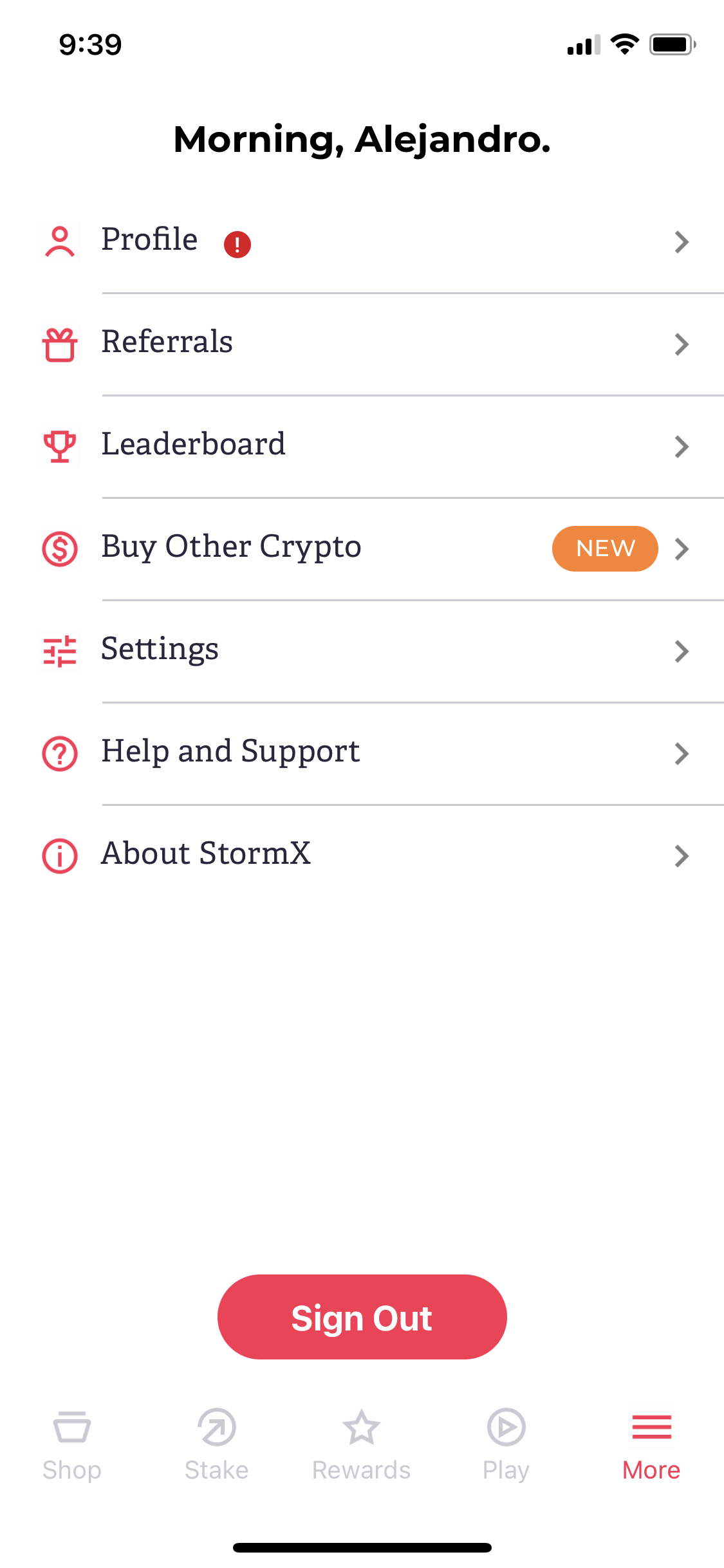The screenshot captures a mobile phone screen with a white background. Positioned in the top-left corner is the time, displayed in black font as "9:39." On the top-right corner, a series of icons indicate the mobile signal, Wi-Fi connection, and battery level. Directly beneath these icons, a bold black greeting reads, "Morning, Alejandro."

The main section of the screen features a vertical list of links, each accompanied by a right-pointing arrow indicating they are clickable. The links are as follows:

1. Profile
2. Referrals
3. Leaderboard
4. Buy Other Crypto
5. Settings
6. Help and Support
7. About StormX

At the bottom of this list, there is a prominent red oval button with white text that reads "Sign Out."

Below the sign-out button, five grayed-out icons are aligned horizontally:

1. Shop
2. Stake
3. Rewards
4. Play
5. More

A thin black line is present at the very bottom of the screen, separating the icons from the rest of the interface.